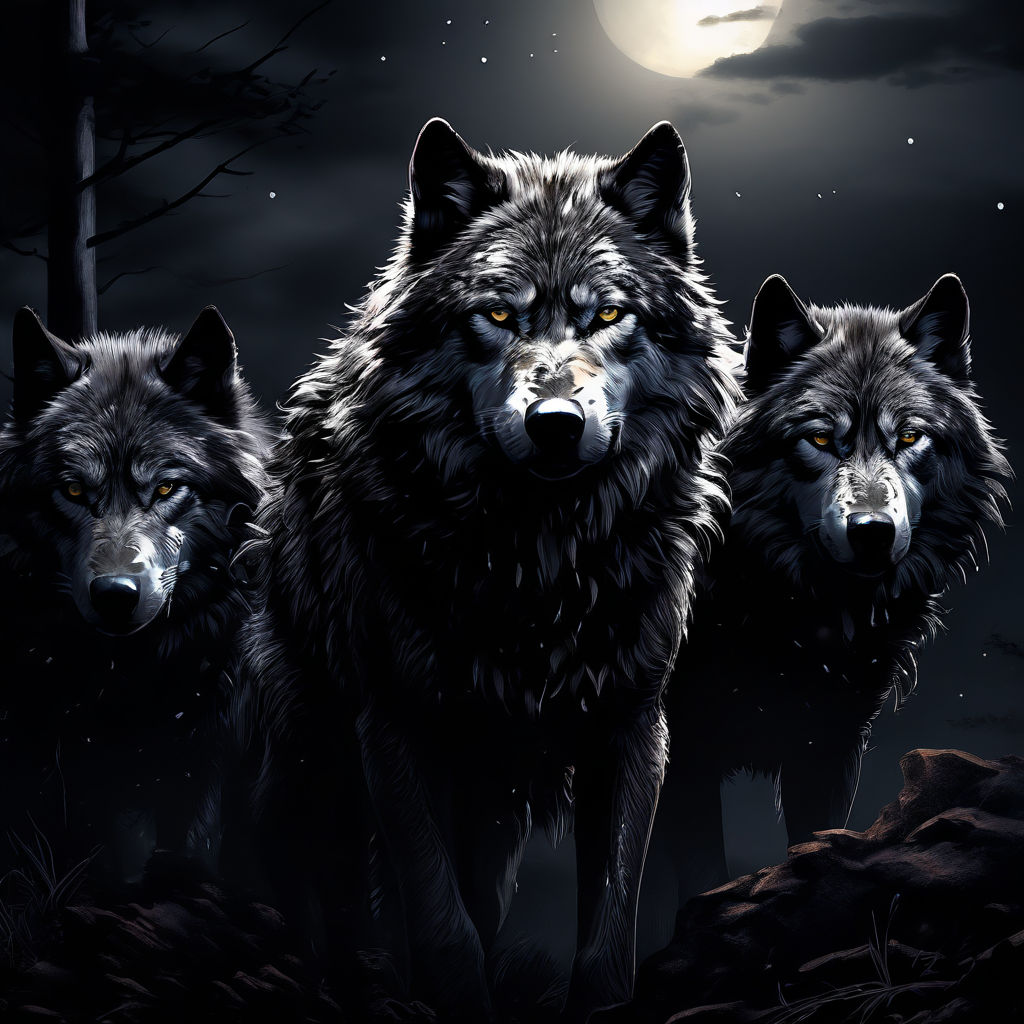The image is a wide vertical, highly detailed, cartoon or computer-generated depiction of a nighttime wilderness scene featuring three wolves. The background showcases a night sky with numerous stars scattered across the black expanse, and a bright full moon partly obscured by wispy dark clouds. To the upper left, a barren tree with black branches reaches into the scene, adding to the nocturnal ambiance.

In the foreground, three wolves stand on rocky ground interspersed with patches of grass. The closest wolf, centered in the image and likely the alpha, stares intently ahead with piercing yellow eyes. Its shaggy fur is predominantly gray with lighter streaks, prominently around the nose and head, possibly reflecting the moonlight above. Upright, pointed ears and black legs complete its formidable appearance. Flanking the alpha, the other two wolves are partially visible—a mere outline of their fur and pointed ears on the left and right edges of the picture, suggesting a pack formation. Their similar features imply they belong to the same group, guarding their territory under the eerie glow of the moonlit sky.